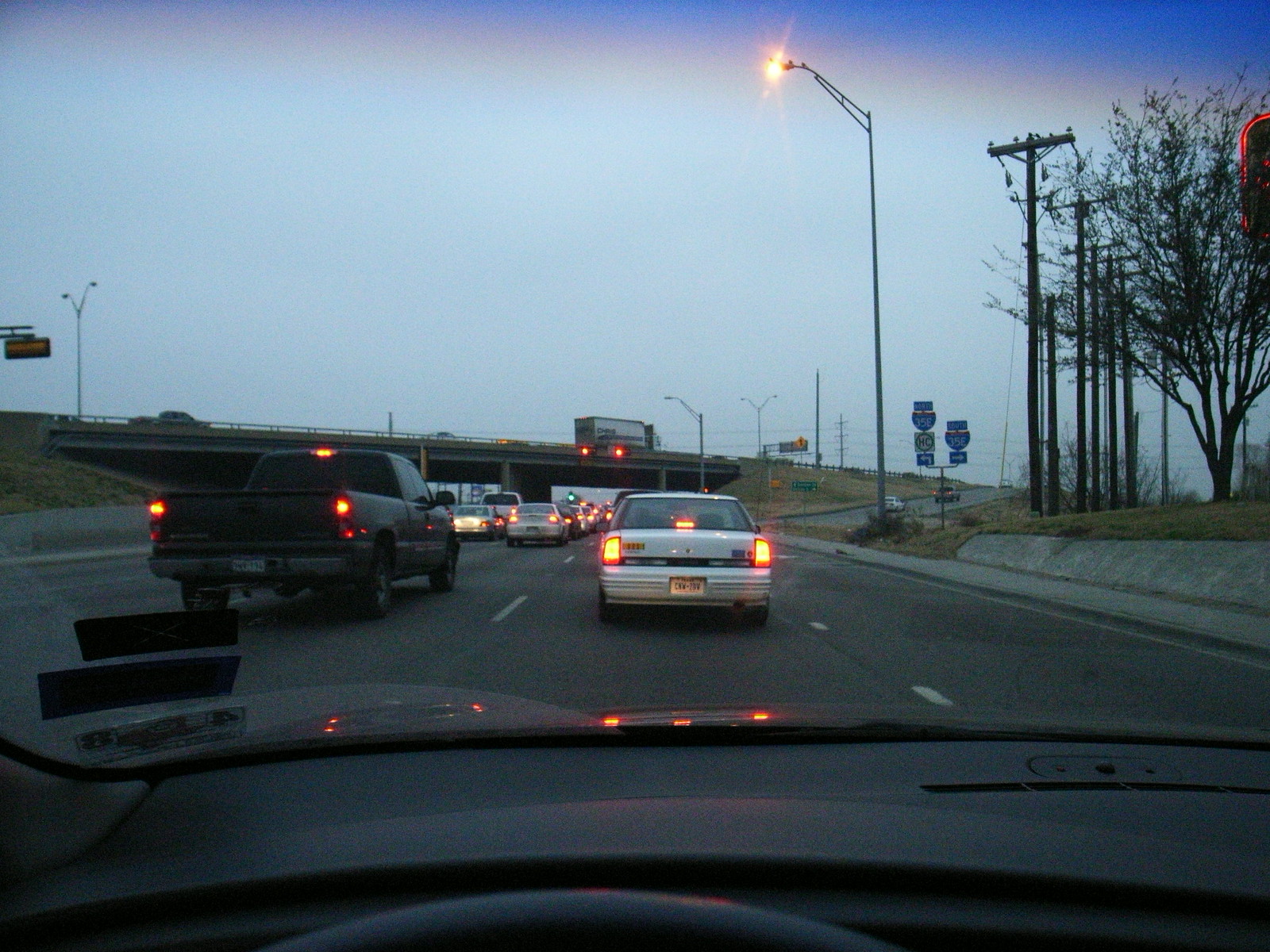The photograph captures a moment either at dawn or dusk, characterized by dim, muted lighting that bathes the scene in a light, hazy gray tone. The image is framed horizontally, focusing on an exterior view through the driver's side windshield. In the background, the sky is overcast, devoid of any discernible clouds, adding to the overall grayness. The foreground is dominated by multi-lane traffic, where every vehicle has its brake lights glowing a stark red against the dim surroundings. Approximately in the center of the frame, an overpass stretches horizontally from left to right. On this overpass, a large semi-trailer is prominently visible. Additionally, traffic lights meant for the vehicles below the overpass are in clear view, glowing red and contributing to the stationary ambiance of the scene.